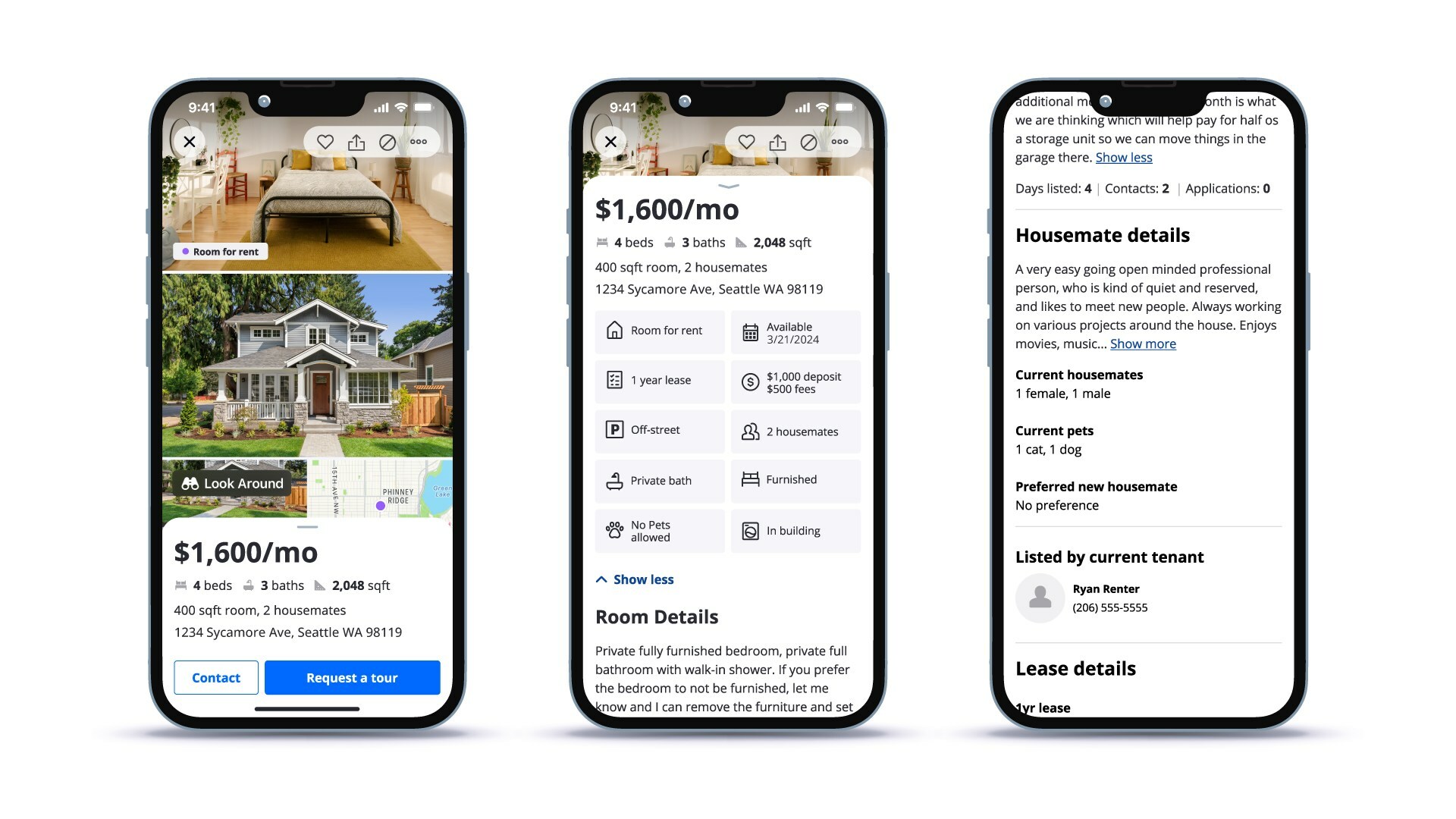Three smartphones display consecutive sections of a real estate property website, illustrating the scrolling motion as the webpage is navigated downward. The first phone on the left showcases the top portion of the site, featuring a detailed photo of a bedroom, followed by an exterior shot of a house. Just below the images, the rental price is prominently listed as $1600 per month. The middle phone captures the subsequent section of the site, providing a seamless continuation of the webpage content. The third phone on the right further extends the view, completing the visual journey through the property listing's details. Each device collectively offers a coherent, progressive glimpse into the real estate website.